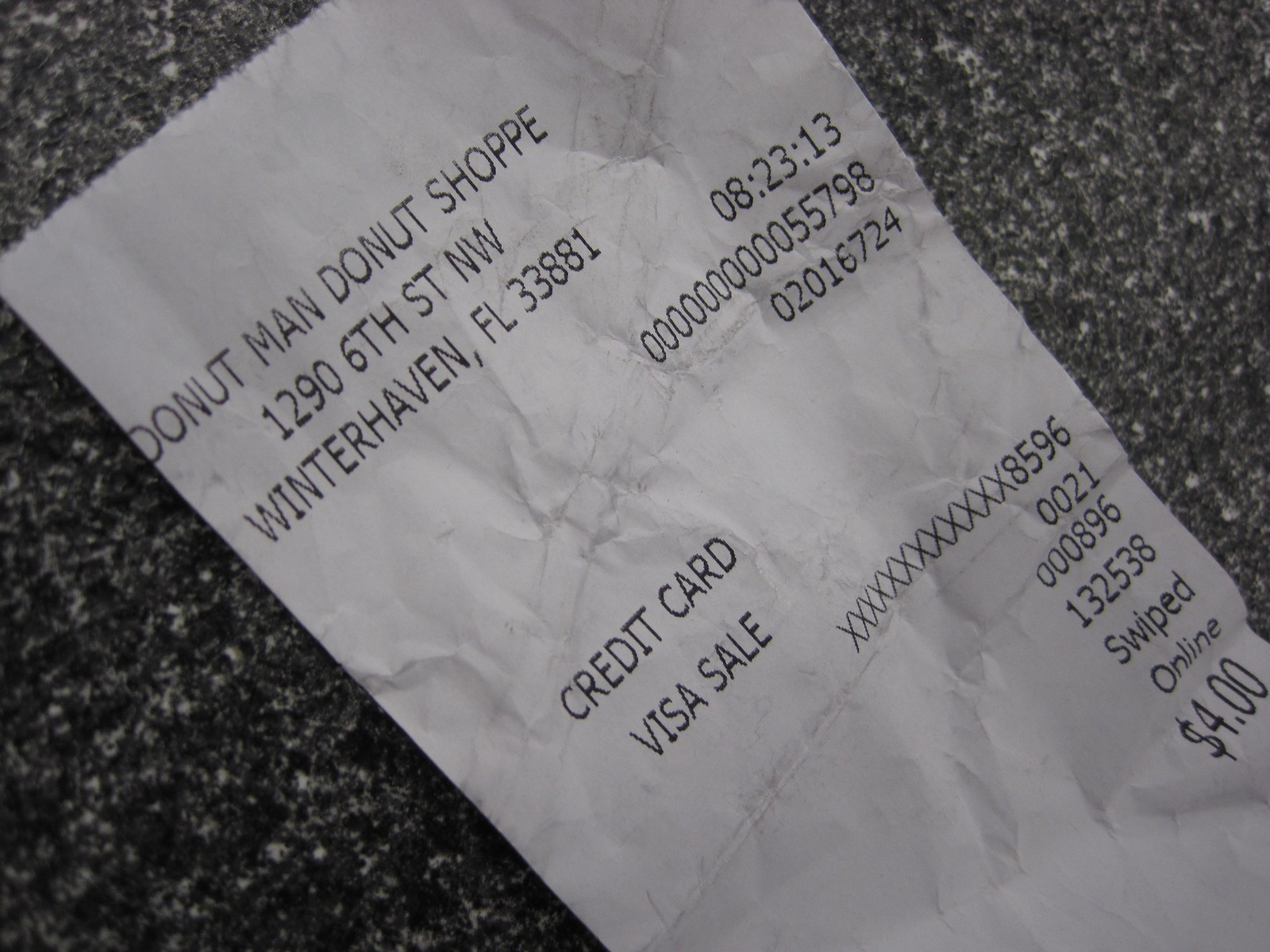This detailed image captures a worn and slightly smudged receipt from Donut Man Donut Shop, located at 1296th Street Northwest, Winter Haven, Florida, 33881. The receipt, printed on standard white receipt paper, shows a total charge of $4 for a credit card Visa sale. The top of the receipt prominently displays "Donut Man Donut Shop" followed by the address. To the right, the transaction time is recorded as 08:23 and 13 seconds. Below this information, a series of identifying numbers are listed: 000000-55798-020-16724. On the left side, the receipt notes "credit card visa sale" and further down, the credit card details are partially masked with a series of X's followed by the last four digits, 8596. Additional sequential numbers—0021, 000896, 132538—are listed with indications of the transaction being "Swiped" and conducted "Online." The background of the photograph is a distinctive stone surface with a pattern of alternating gray and white dots, adding a textured contrast to the smooth white paper of the receipt.